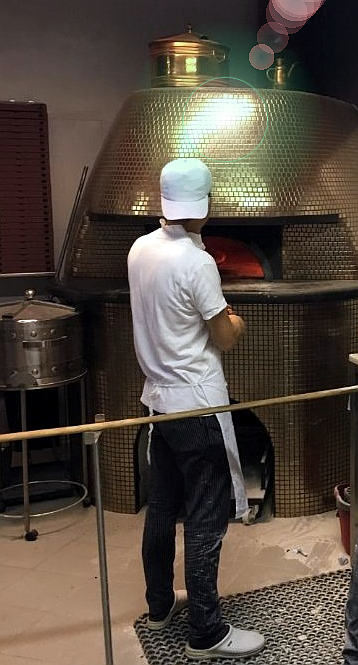In this photograph, we see a restaurant worker standing with his back to the camera in front of a large, modern, shiny, silver pizza oven that emits an orange glow, indicating it is in use. The worker is wearing a backward white baseball hat, a white collared short-sleeve shirt with a popped collar, a white apron, black or dark blue pants speckled with flour, white or gray Croc-like shoes, and black socks. He appears to be holding a pizza peel, positioning something into or taking something out of the oven, though the food item is not visible. To the worker's left, there's a small, circular metal machine mounted on thin legs, resembling a birdhouse on a stool with wheels. The floor consists of tiles and features a black, grate-like mat beneath the worker, possibly scattered with white flour. There's also a brown board situated somewhere on the worker’s left side.